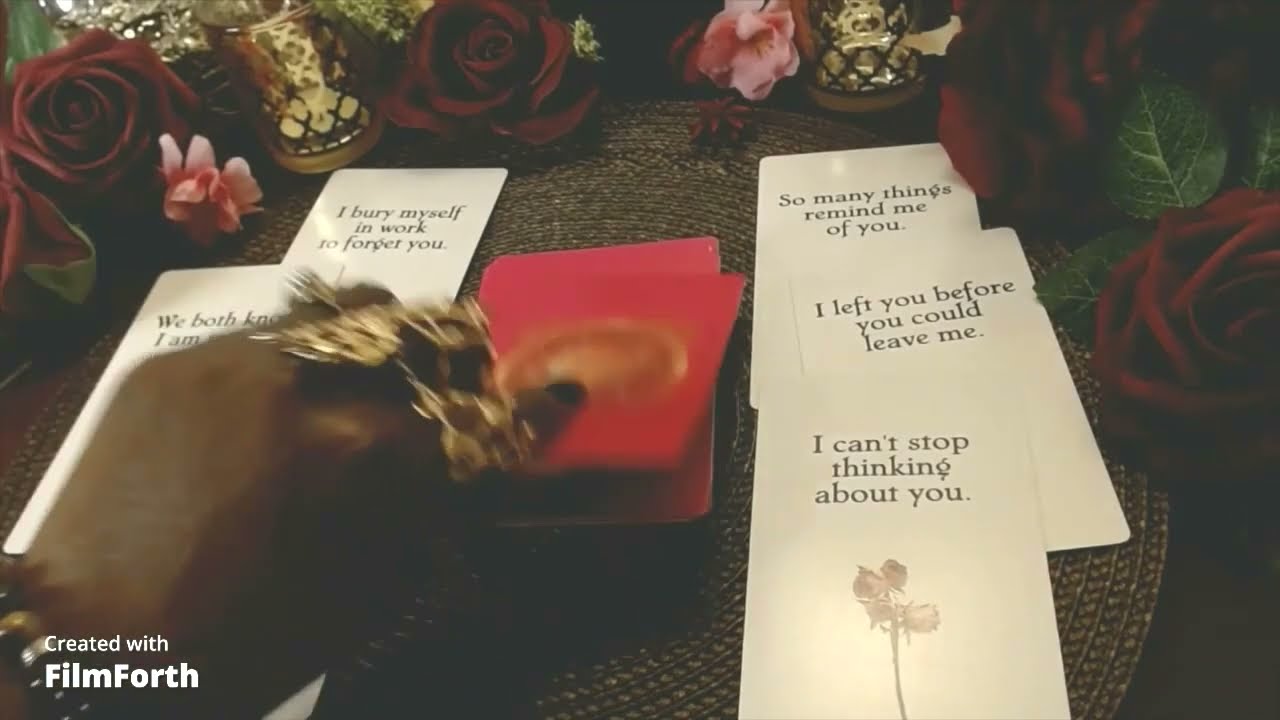In this close-up image, we see a beautifully adorned table featuring a collection of red and white cards. The table is surrounded by a stunning arrangement of red roses and pink flowers forming a semicircle. Amidst the flowers, especially in the upper left-hand corner, a gold vase is visible. At the center of the table lies a pile of red cards, characterized by a blurred gold circular logo. Emerging from the lower left corner, a black hand adorned with multiple gold rings reaches to pick up a card from the pile. To the left of the hand, two white-background cards are flipped over, with one card bearing the message: "I bury myself in work to forget you." On the right-hand side, another pile of three cards displays the phrases: "So many things remind me of you," "I left you before you could leave me," and "I can't stop thinking about you." The image also includes a watermark in the bottom left corner that reads, "created with Filmforth." This first-person perspective suggests an intimate moment, possibly involving a tarot card reading or a card game.